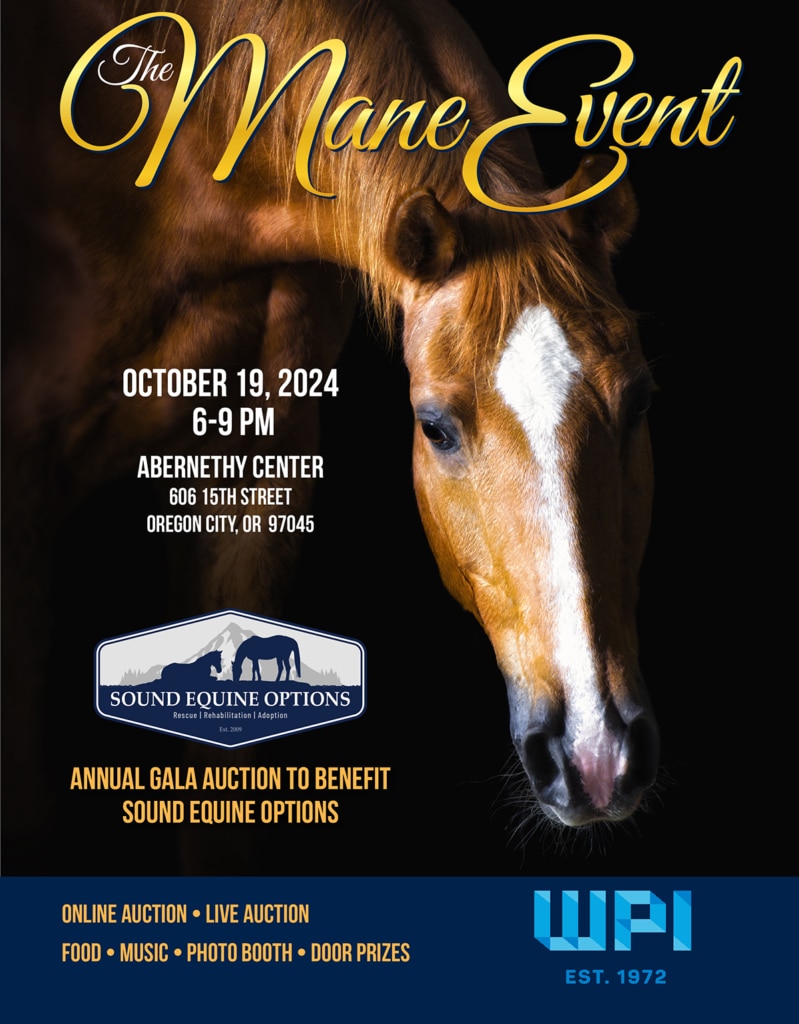The photograph is a visually striking poster for an upcoming event, dominated by the image of a brown horse with a distinctive white stripe running vertically down its face. The horse's black eyes and nostrils stand out against its well-defined features. Overlaid on this engaging backdrop is elegant gold cursive text announcing "The Mane Event," cleverly playing on the word 'mane.' Further details are provided in white text, stating that the event will take place on October 19th, 2024, from 6 to 9 p.m. at the Abernethy Center, located at 606 15th Street, Oregon City, OR 97045. A hexagonal logo featuring the outline of two horses is prominently displayed, identifying the organizer as Sound Equine Options, an organization committed to rescue, rehabilitation, and adoption. Additional information at the bottom of the poster highlights that this annual gala auction is to benefit Sound Equine Options, and promises a lively evening with an online auction, live auction, food, music, a photo booth, and door prizes.